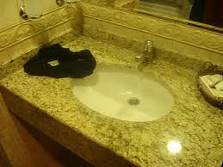A detailed image of a bathroom countertop showcases a small, oval-shaped, white porcelain sink adorned with a sleek silver faucet. The countertop is crafted from a light beige or brown marble, seamlessly blending with the similarly colored wall. Decorative crown molding encircles the sink, adding an elegant touch to the bathroom decor. To the left of the sink, a piece of black fabric—possibly an item of clothing—rests, with part of it slightly draping into the sink's rim. Adjacent to this fabric is a metal hook affixed to the wall, likely intended for a washcloth or towel. Behind the faucet, a small section of the mirror is partially visible, although its reflection is not discernible in the image. On the right side of the sink, a small basket is placed on the countertop, presumably for holding soap or hand towels, though its contents are not clearly defined.